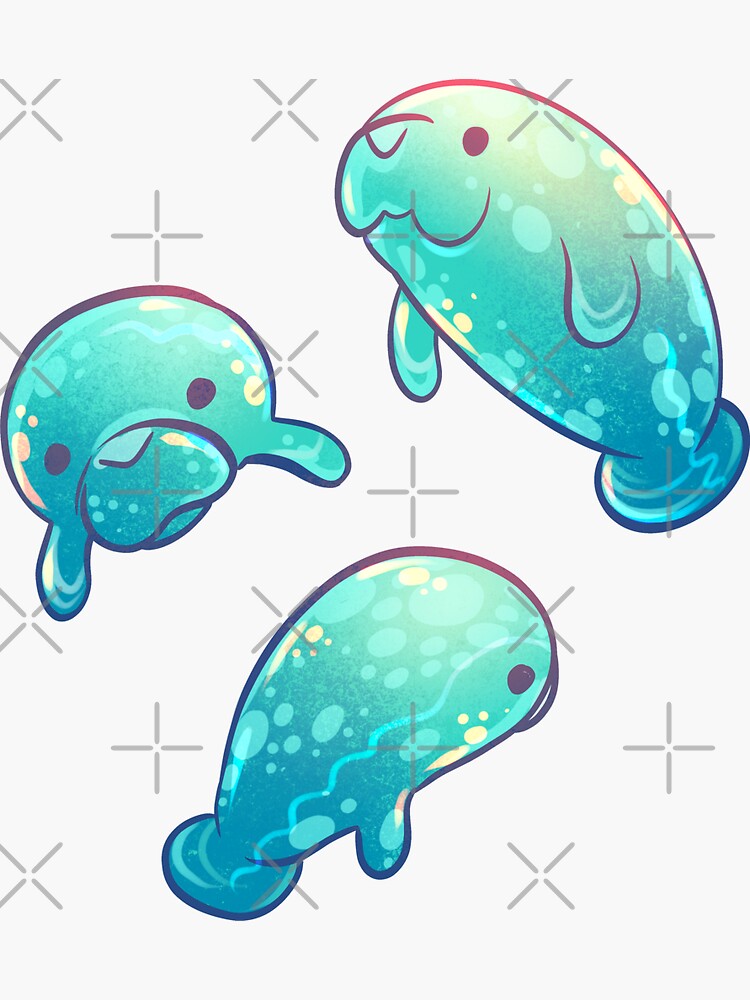This image features a detailed, cartoonish clip art of three sea creatures, which are likely manatees or sea otters, illustrated in a whimsical, teal-green hue. These adorable animals are drawn in a cute, cartoon style, each with beady black eyes, an upside-down triangle nose, and a round body shape. The manatees are adorned with various markings, including white bubble-like circles and small yellow dots scattered around their bodies.

The composition places each manatee in a distinct position: one in the upper right shows its left side and underneath, appearing to angle upward; another on the middle left edge faces forward, showing only its face and flippers; the third, located at the bottom center, is depicted from the right side, with a squiggly line running down its back.

The background adds to the playful theme with medium-sized x's and plus signs arranged in a repeating pattern throughout the image. There are rows of three plus signs alternating with rows of three x signs, providing a vibrant setting for these charming creatures.